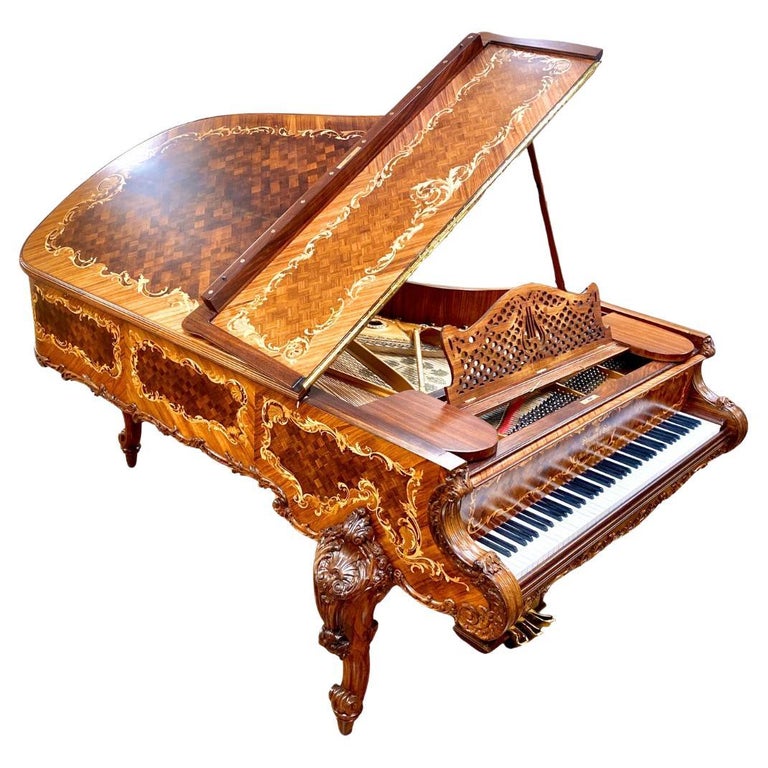This is a detailed and ornate antique grand piano, likely from the 1800s, crafted predominantly from dark mahogany wood with intricate design elements. The piano features a variety of light and dark brown wood details, including inlaid leather and swirling scroll work, which together create a luxurious and high-quality appearance. The top of the piano can be propped open using a wooden pole, revealing the inner workings and strings. The piano is supported by three Queen Anne Cabriole carved legs, enhancing its majestic presentation. On the top lid, which is able to fold down and latch securely, there is a diagonal checkerboard pattern framed by a fancy border, adding to its elaborate aesthetic. The surface is adorned with elaborate curls and filigree. Measuring approximately 10 feet long, 6 feet wide, and 2 to 3 feet tall, the grand piano includes standard ebony and ivory keys. The photograph, professionally taken and edited against a plain white background, highlights the piano's elaborate designs, such as squares, swirls, and various stripes, demonstrating its historical and artistic value.